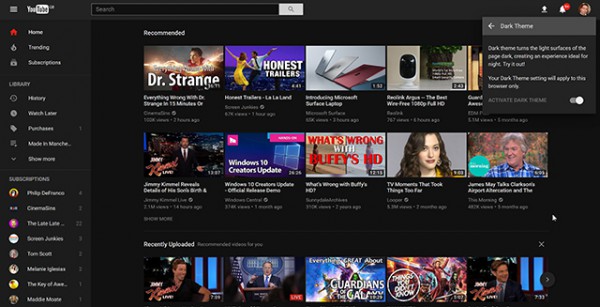In the given image, it is clear that this is a screenshot of a YouTube interface.

In the top left corner, there's a hamburger menu, followed by the YouTube logo and a search bar prominently placed adjacent to it. A white notification bell icon sits to the right, indicating the user’s notification alerts. The entire interface is marked by its signature clean, white design.

On the left side of the screen, there's a vertical navigation panel featuring icons and text for different sections: Home, Trending, Subscriptions, Library, History, Watch Later, Purchases, and a section for more options. Under the Subscriptions section, some of the visible channels include "DeFranco," "Cinefix," "Smosh," "Late Late Show with James Corden," and "Scott Manley."

In the center of the screen, the primary content area showcases various video thumbnails. The top video thumbnail is titled "Everything Wrong with Doctor Strange in 11 Minutes" from CinemaSins. Adjacent to it is an Honest Trailers video. Another prominent thumbnail promotes the "Microsoft Surface Laptop" featuring Jimmy Kimmel, showcasing one million views. 

Additional video thumbnails displayed include a "Windows 10 Creators Update Official Release Demo," and "Buffy's TV Moments That Took Things Too Far."

This detailed caption encapsulates the user interface elements and video content visible in the YouTube screenshot.